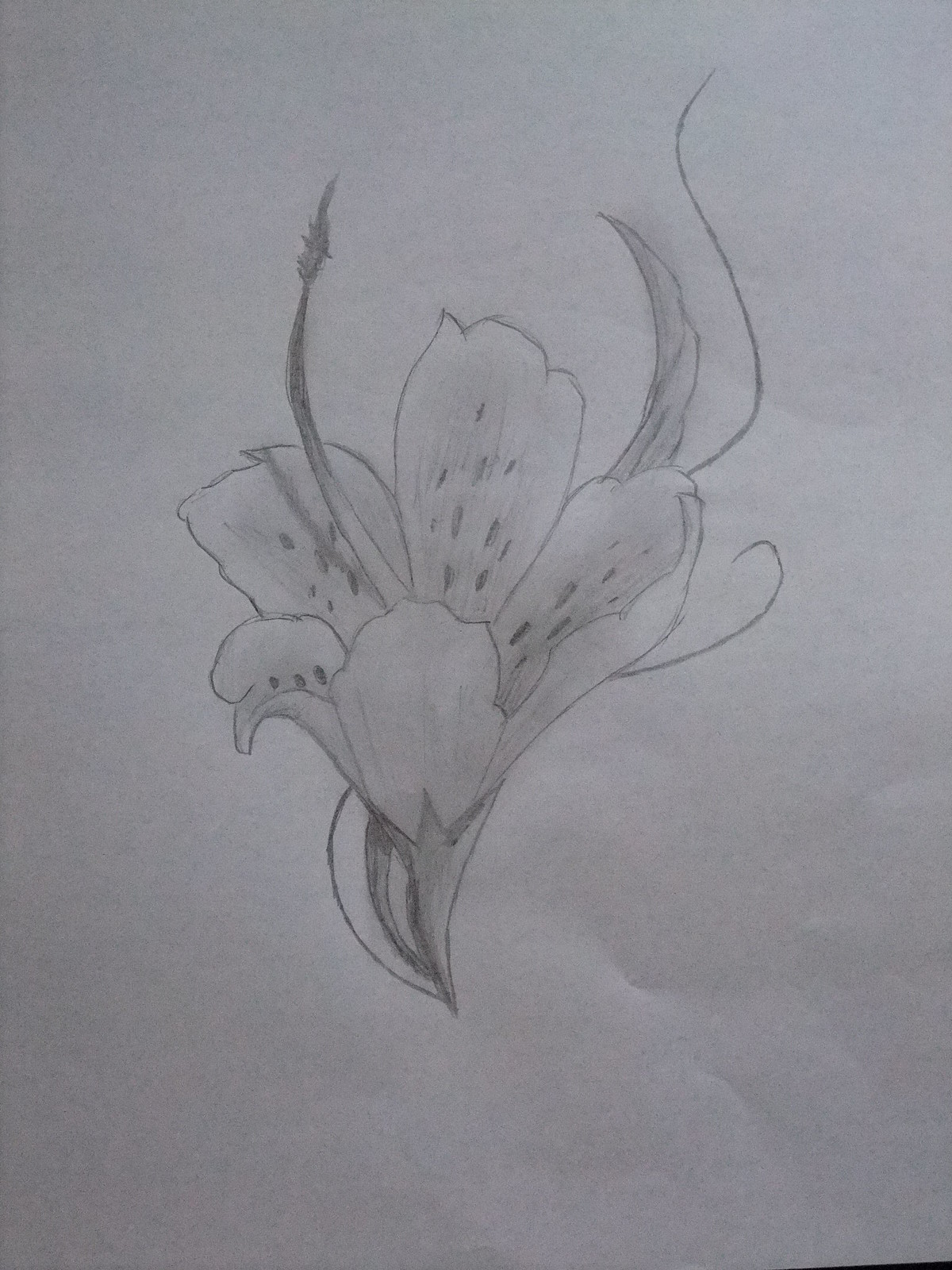This black and white photograph captures a detailed pencil drawing on white paper, presenting the image of an orchid-like flower, potentially a lily. The composition is in portrait mode, with the flower taking center stage, leading the viewer’s eye from the base to the top as the bloom trails off the upper edge of the paper. The flower itself consists of a central bulge from which five petals emanate, each displaying intricate markings and tiny dot-like details on their inner sides. The side view obscures the complete center of the flower due to overlapping petals, enhancing the three-dimensional appearance of the drawing. From the core of the flower, slender sepals curve upwards, contributing to the naturalistic portrayal. Although rendered in pencil shades of gray, the precision in lines and texture underscores the detailed beauty of the flower, making up for the absence of color by highlighting the structural elegance typically enhanced by the natural hues of orchids.